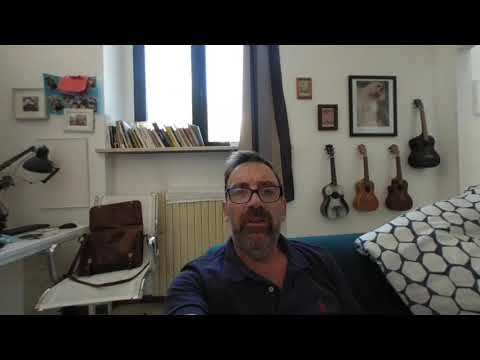The photograph features a middle-aged man with dark brown, somewhat salt-and-pepper hair, sporting glasses, a mustache, and a beard. He is seated on a blue soft fabric couch, taking a selfie. He is wearing a navy blue, short-sleeved polo shirt with the buttons undone, a distinctive feature being the red Polo Ralph Lauren logo on the chest. Next to him is a neatly folded blanket covered with white hexagons and black lines. The man is positioned in a room with a variety of details: behind him, a white wall adorned with multiple picture frames and four ukuleles in different colors—white and black, brown, dark brown, and black. At the center of the wall is a tan radiator with a white cloth on top. Above the radiator is a two-pane window with a black frame and a black curtain pulled open to the right, revealing a shelf on the windowsill filled with books. To the left, there is a white chair in front of a desk with a lamp, holding an open brown leather satchel. The room is filled with natural light streaming through the uncovered part of the window.